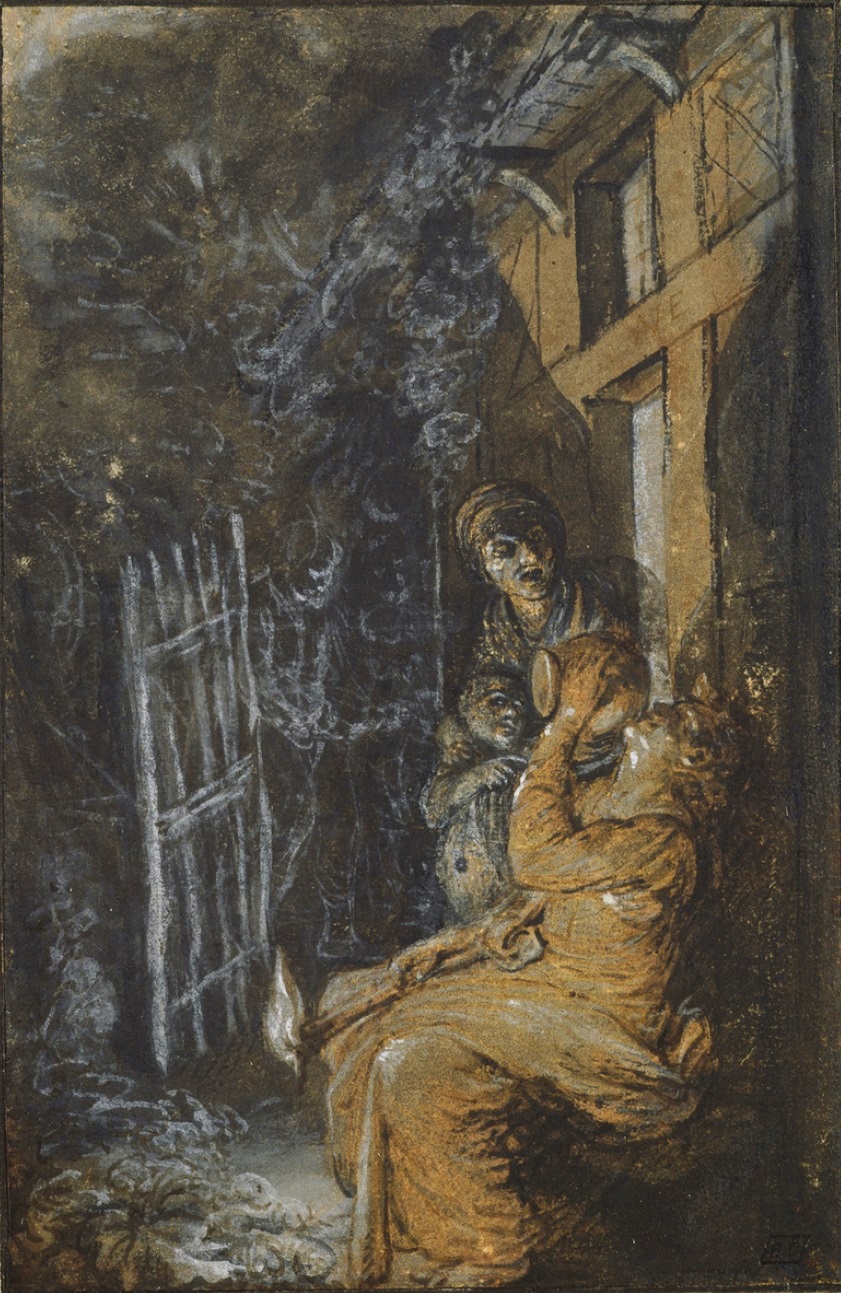The image depicts a detailed, hand-painted scene set outdoors in front of a wooden home, likely representing a period from the 1930s or 1940s. Dominating the bottom right corner, a woman sits on a bench, dressed in a long, traditional gown, holding a clay jug from which she appears to be either drinking or pouring water onto herself. Nearby, to the right, a man and a child stand in the doorway, watching her intently. The setting includes a wooden picket fence, and the overall atmosphere of the composition is enhanced by swirling white fog or smoke in the corners, adding an ethereal touch. The painting's color palette consists of earth tones such as brown, beige, black, and white, contributing to its vintage and somber mood.